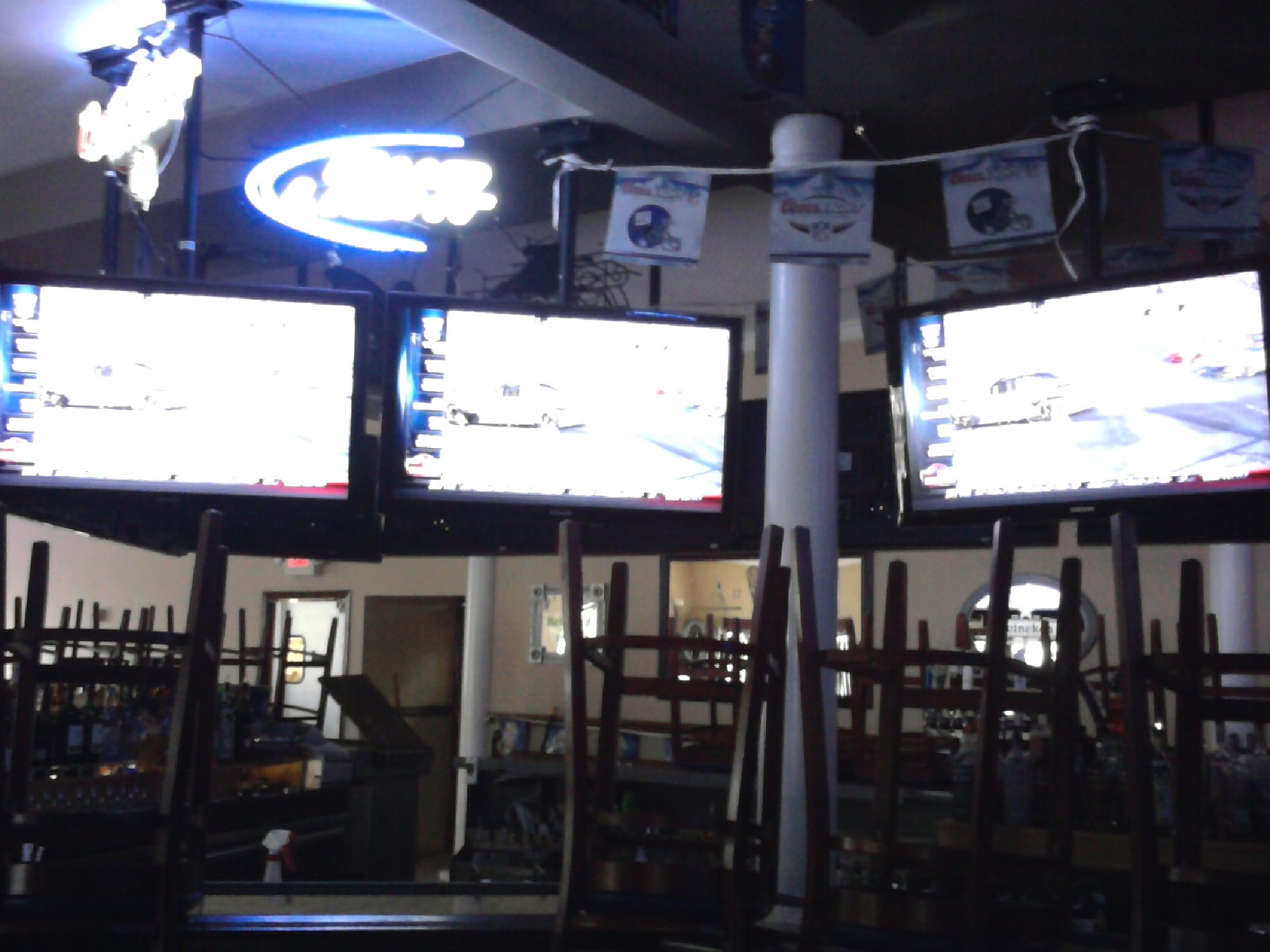This extremely blurry photograph likely depicts the interior of a sports bar near closing time. The lighting in the image is overly bright, obscuring many details. In the background, three large TVs are mounted side by side, possibly displaying a NASCAR race on ESPN, although the brightness makes the content difficult to discern. The bar area itself is cluttered with all the chairs placed upside down on the tables and counters, indicative of the end of service as staff prepare to clean up. On the upper left side of the photo, there's a neon Bud Light sign, identifiable more by its logo than legibility due to the intense exposure. Additionally, a central white column is adorned with a banner featuring football helmets and another unidentifiable logo. Mirrors on the walls add to the reflective chaos of the brightly lit room, contributing to the overall garish and indistinct ambiance.